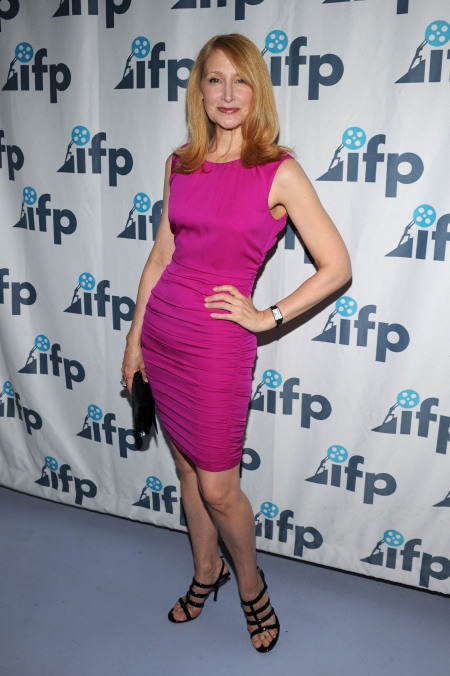A woman, possibly in her 40s, poses confidently for a photograph in front of an official backdrop at an event, likely film-related due to the recurrent logo. The background is white with a repeating emblem that includes a dark gray "IFP" and a blue film reel sitting atop the "I," which is being pushed upward by a cartoon-like human figure on a triangular incline. She stands out in a vibrant, dark pink dress that fits tightly and reaches her knee. Her footwear consists of stylish black strappy sandals with heels. Accentuating her outfit, she carries a black purse in her right hand and wears a watch on her left wrist. With long auburn hair cascading to her shoulders and a subtle peach tint on her lips, she strikes a poised stance with her left hand resting on her hip, looking directly into the camera. The floor beneath her is gray, completing the polished scene.